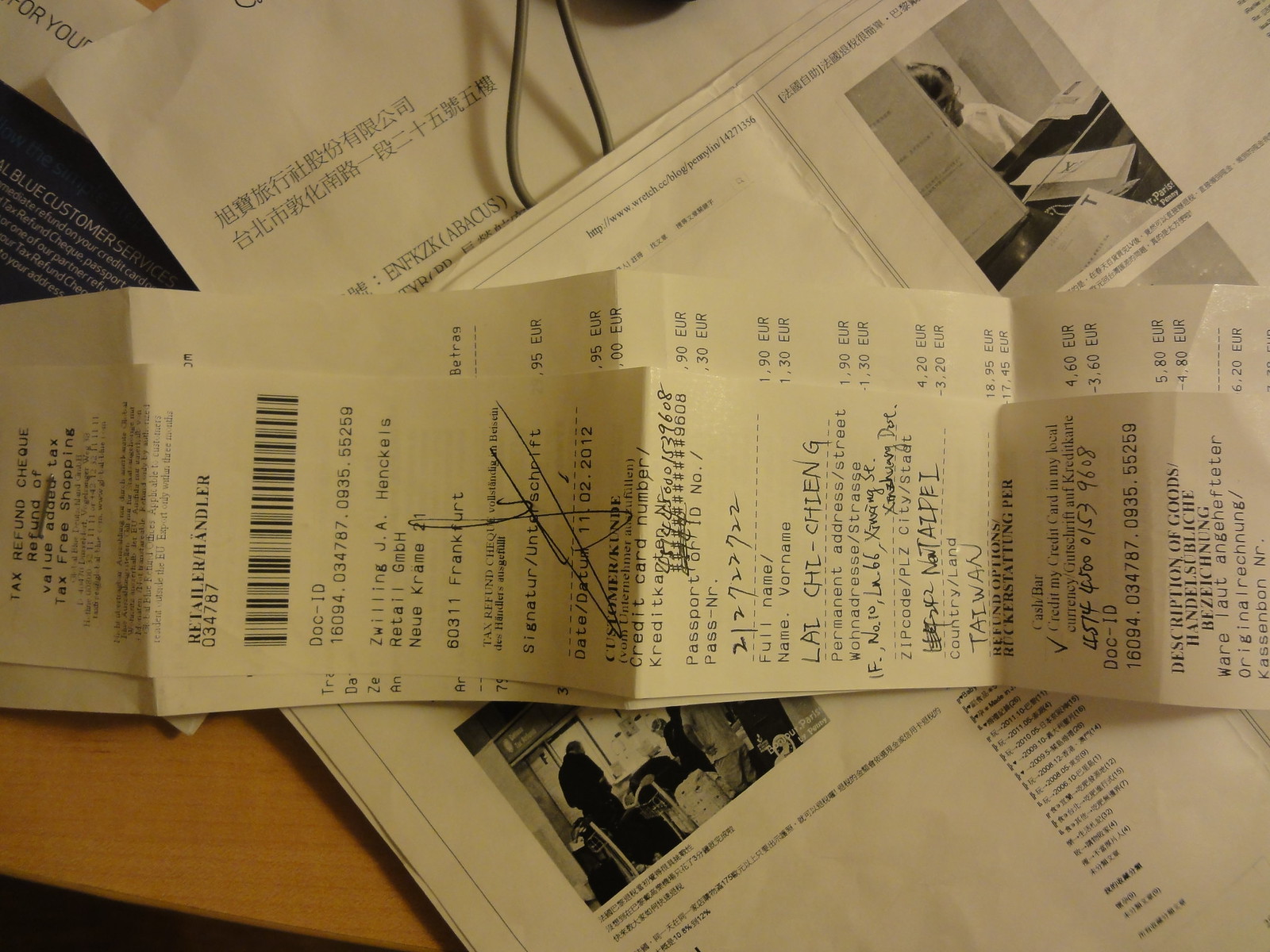A detailed caption for the image: Captured horizontally, the image features a receipt situated on a table. The receipt is from Taiwan, as indicated by the mention of "Taiwan" on it. The table is cluttered with various papers displaying pictures and Chinese characters. The receipt includes a barcode and a plethora of information, including a date of "2-22." A name, pronounced as Lai Chi Chien Chien, is also visible on the receipt.